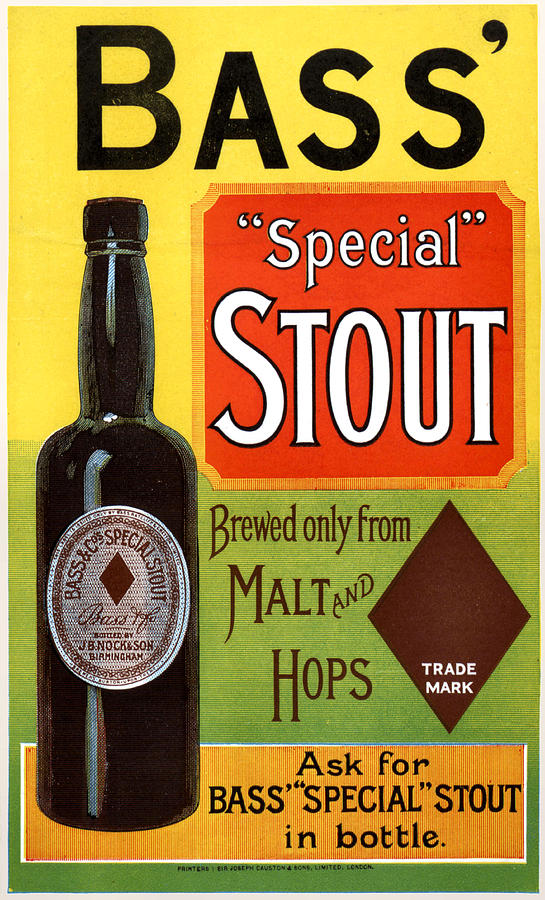This image is a detailed vintage advertisement for Bass's Special Stout, likely from the 1950s. The ad features a colorful background, with the top half bathed in yellow and transitioning to light green in the lower half, further decorated with an orange banner. At the very top in black text, it reads 'Bass'. Right below this, on the right side, there's a red box outlined in orange, containing white text that says "Special Stout." Dominating the left side of the ad, a large dark brown bottle of Bass Special Stout extends upward from the green area. The bottle features an elliptical label with 'Bass & Company's Special Stout' and a rhombus-shaped logo that reads 'Trademark'.

In the middle, across the green area, the text proclaims, "Brewed only from malt and hops." At the bottom, an orange banner spans the width, inscribed with the black text, "Ask for Bass Special Stout in Bottle." Additionally, there is a small signature in the orange section stating, "Bottled by J.B. Knock & Son, Birmingham." This advertisement encapsulates the essence of a bygone era with its colorful design and detailed branding.